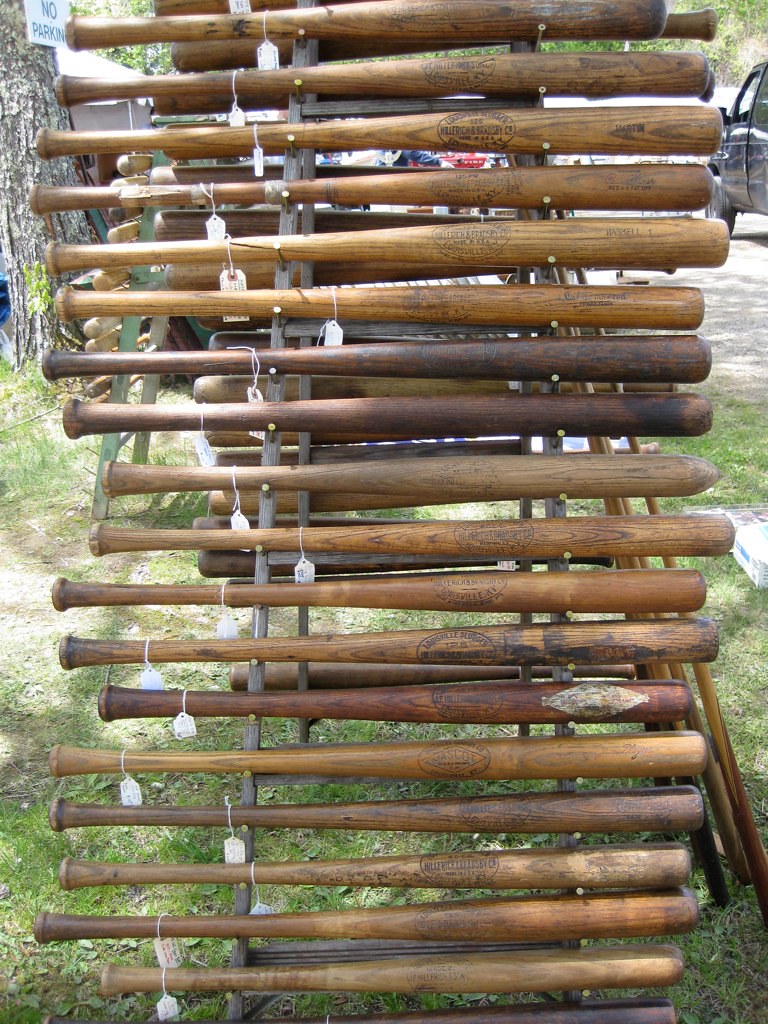This color photograph depicts a collection of wooden baseball bats arranged horizontally on a two-sided A-frame metal rack situated outdoors on a grassy area. The bats, which vary in size and range in color from dark to light brown, occupy roughly 95% of the image's width and the entire height. Each bat features a small tag near the handle, indicating they might be part of a retail display. Sunlight filters through the middle of the frame, offering a natural glow. In the background, on the upper right, there's a glimpse of a greyish-black car on a road, while to the far left, a grey tree trunk is visible with a "no parking" sign and a nearby tent. Intricate details such as a small patch of blue and pink can be seen at the very top between the bats, possibly part of a person. The bats lack distinct markings, with the exception of one that has some unreadable printing, and they appear to be somewhat aged rather than brand new.